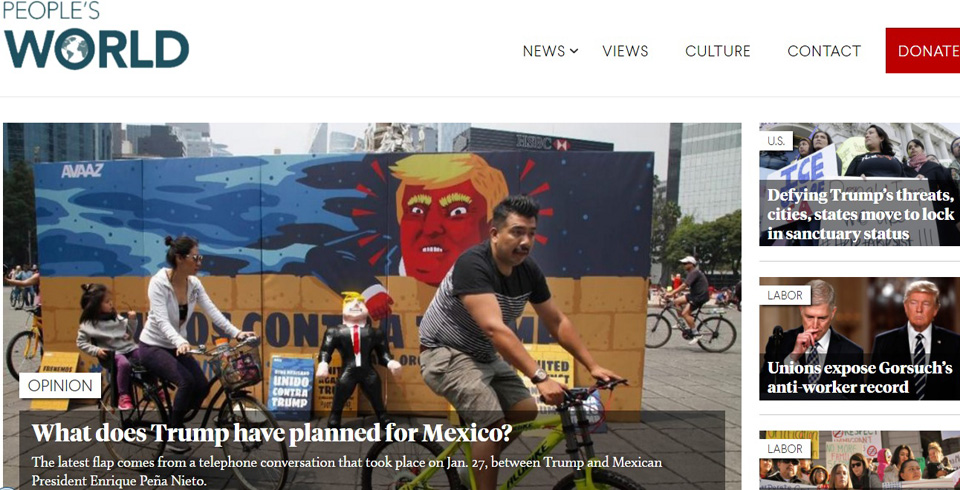The screenshot captures the top corner of a webpage titled "People's World." The logo features the word "People's," with the letter "O" creatively designed as a globe. On the right, there's a menu bar with options labeled: News, Views, Culture, Contact, and Donate. To the left is a vibrant photograph depicting people riding bikes past a mural. The mural is a highly exaggerated caricature of Donald Trump with a bright red face and vivid orange hair and eyebrows, peeking over the top of a wall. Below the mural, there's an inflatable caricature balloon and a sign displaying "UNIDO CONTRA TRUMP." The main headline reads: "Opinion. What does Trump have planned for Mexico?" This article points to a controversial telephone conversation that occurred on January 27 between Trump and Mexican President Enrique Peña Nieto. To the right of the main article, there are three additional headlines: "Defying Trump's Threats, Cities, States Move to Lock in Sanctuary Status," "Unions Expose Gorsuch's Anti-Worker Record," and a third partially visible headline at the bottom edge of the screenshot. The image contains no animals or airplanes.